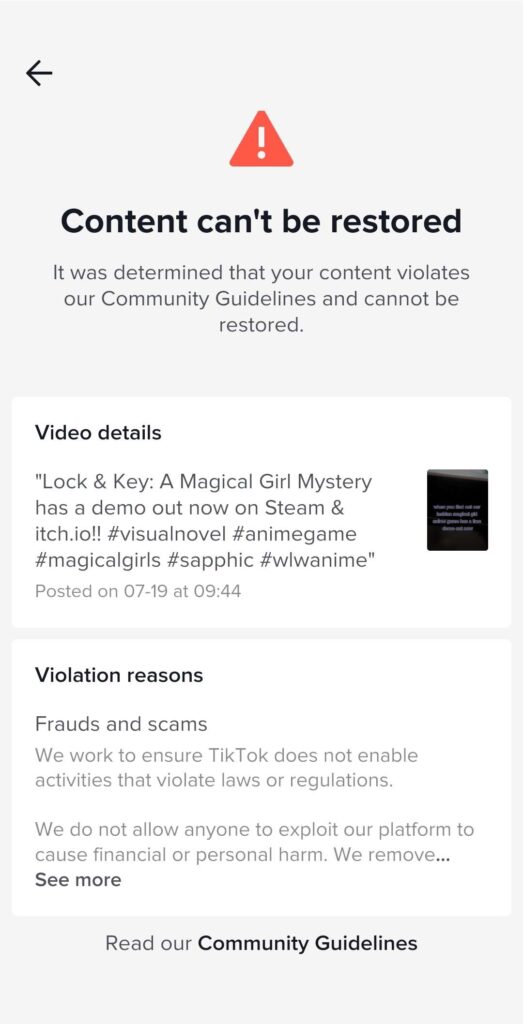This image displays a notification page, likely from the TikTok app. The top of the page features a red header with a white exclamation mark, accompanied by a message stating "Content can't be restored." It further explains that the content was removed for violating the community guidelines.

Below, the section titled "Video Details" shows the title "Locking Key: A Magical Girl Mystery," and notes that a demo is available on Steam and itch.io. Visible hashtags include #VisualNovel, #Anime, #Game, #MagicalGirls, #Sapphic, and #WLWAnime. The post was dated 7/19 at 9:44.

The violation reasons listed are "Frauds and Scams," with a brief explanation: "We work to ensure TikTok does not enable activities that violate laws or regulations. We do not allow anyone to exploit our platform to cause financial or personal harm." However, the explanation is cut off with ellipses and a "See more" button.

At the bottom, there's an option to "Read our Community Guidelines."

The majority of the page has a gray background, white text boxes, and black text, resembling a typical in-app notification on a smartphone.